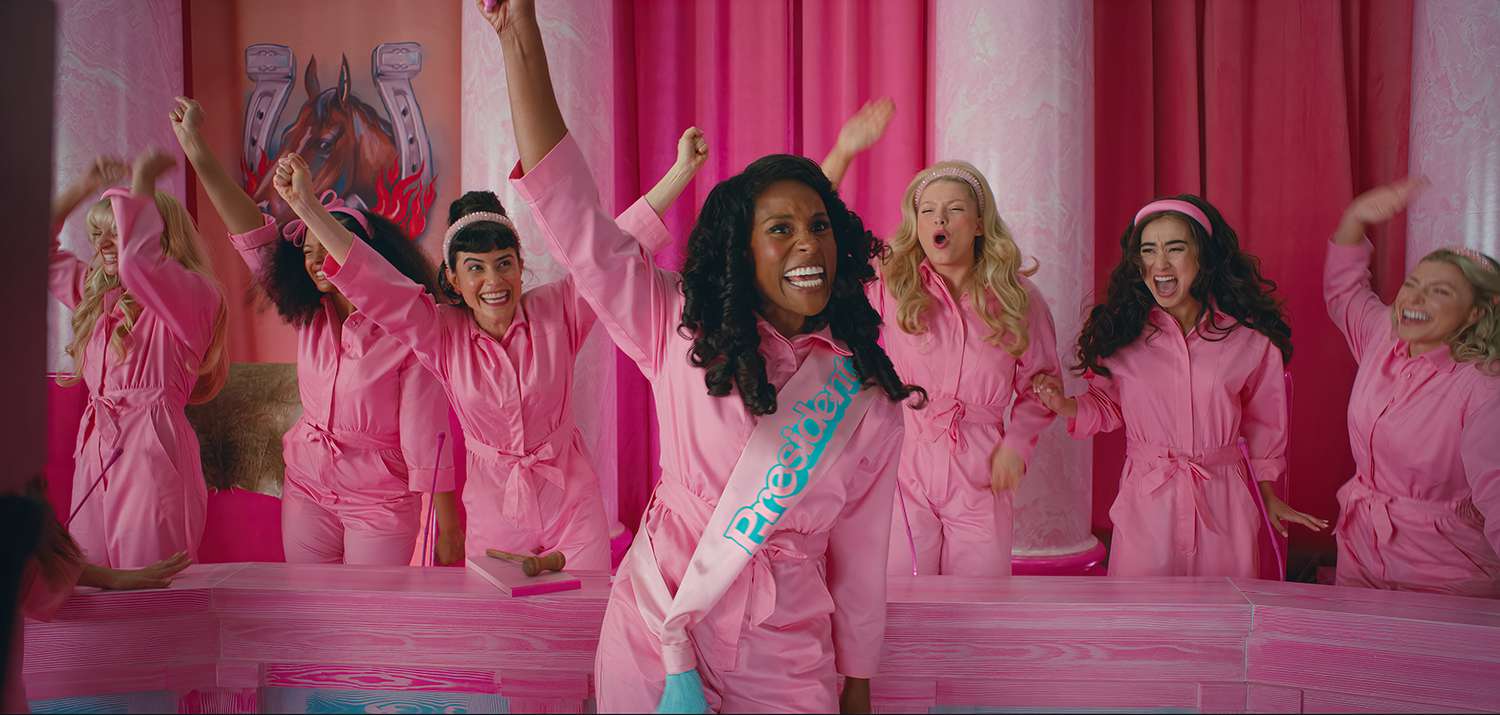In this vibrant scene from the Barbie movie, Issa Rae stands prominently in the foreground, wearing a bright pink jumpsuit and a sash emblazoned with the word "President" in bold blue letters and adorned with blue tassels. Issa Rae, a darker-skinned woman with curly black hair, has her arm raised triumphantly above her head as she celebrates. Surrounding her are six other women, also dressed in matching pink jumpsuits, each with their arms raised in a similar celebratory gesture. The women, a diverse mix of different races with a variety of hair colors ranging from blonde to brunette to black, appear to be in high spirits, some seemingly jumping up and down with joy. The setting is adorned in pink hues, including pink columns and curtains, with a striking mural of a horse emerging from a horseshoe visible in the background. A pink bench is situated behind Issa Rae and the group of cheering women. The image captures a jubilant moment, with smiles and cheers resonating throughout the scene, embodying the quintessential Barbie pink aesthetic.